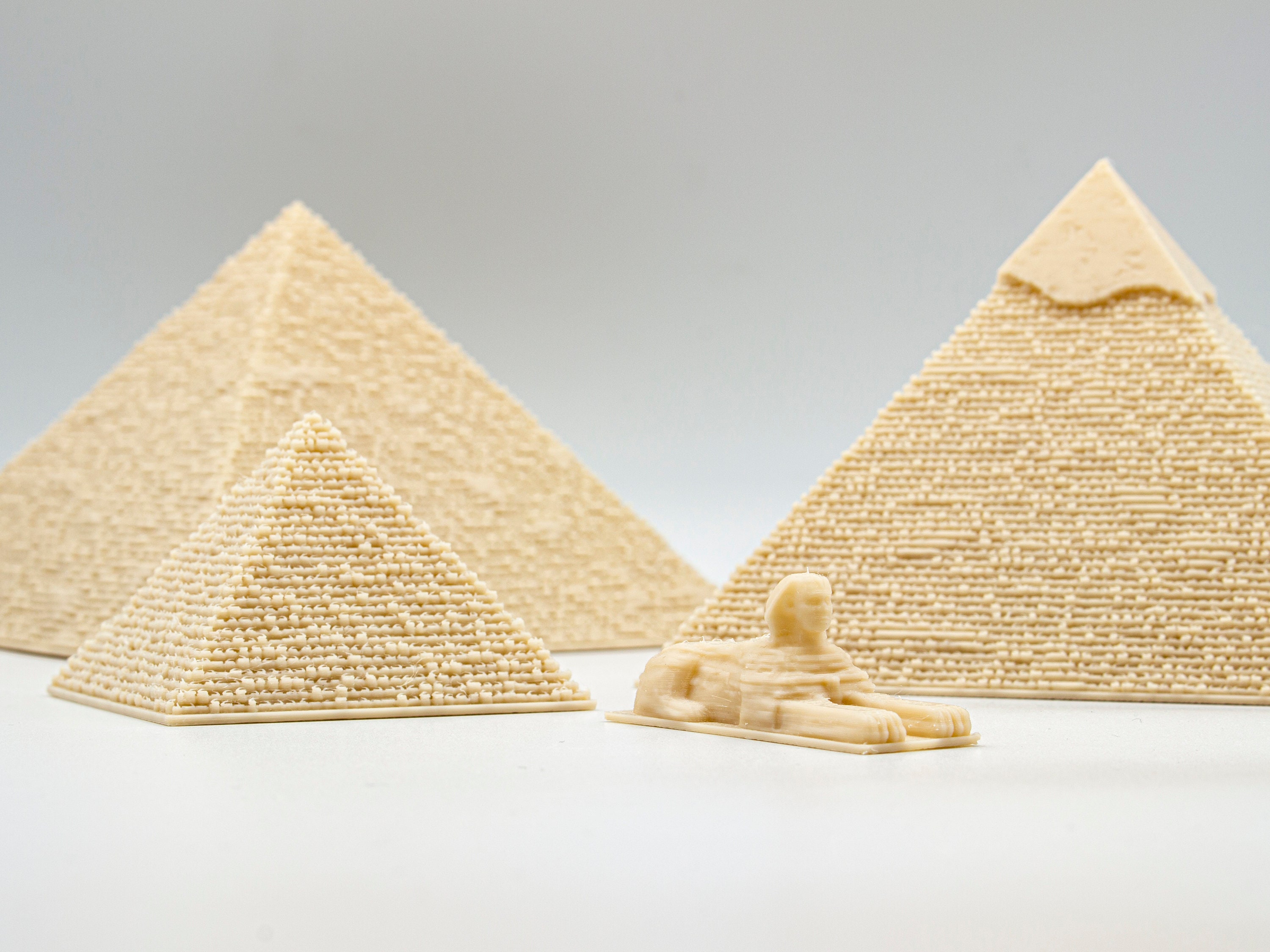This photograph showcases four 3D-printed sculptures replicating iconic Egyptian landmarks, set against a smooth, light gray background and resting on a white surface. The sculptures are all a light beige color, consistent across all pieces. In the foreground lies a small, stoic-looking Sphinx sculpture, with a complete human face, body of a lion, and detailed paws. Positioned behind the Sphinx are three pyramids of varying sizes, reminiscent of the pyramids of Giza. The pyramid on the right side stands out with its smooth, flat apex, while the rest feature a detailed, textured surface resembling layers of small cubes or bricks. The composition highlights the intricate details of the sculptures, offering a visually engaging tribute to ancient Egyptian architecture.